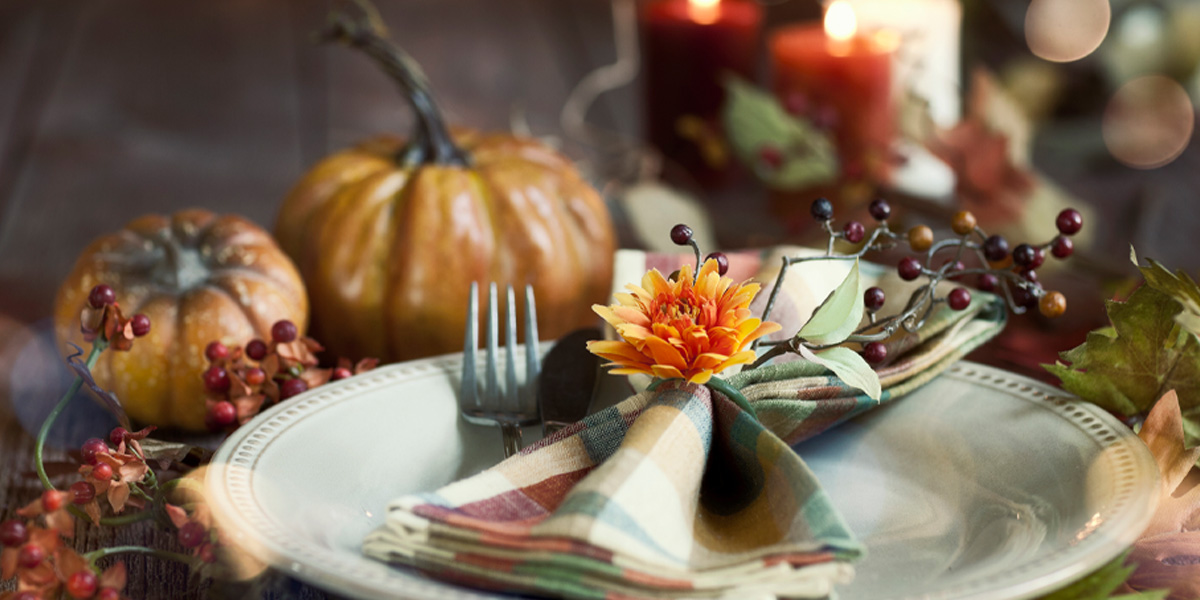In this detailed still-life photograph, capturing an autumnal October ambiance, the focal point is a close-up of an elegantly set fine china plate on a rustic wooden table. The plate, white with gold dots around its rim, is adorned with a folded napkin featuring a muted palette of whites, beiges, and subdued stripes of greens, blues, and reds. This napkin is intricately tied together with a cloth ring, topped with a striking orange flower, and embellished with a sprig of tiny berries. The silverware, comprising a fork and a butter knife, rests neatly on the plate to the left of the napkin.

Surrounding the plate, additional sprigs of berries and clusters of deciduous leaves contribute to the decorative ensemble. In the background, partially out of focus, three lit candles—one white, one light red, and one darker red—cast a warm, inviting glow. Additionally, small pumpkins, prominently orange with varying stalk sizes, enhance the seasonal feel. The overall composition is bathed in natural light, possibly streaming in golden rays, which highlights the textures and details, creating an inviting, elegant, and festive scene reminiscent of a cozy autumn day.